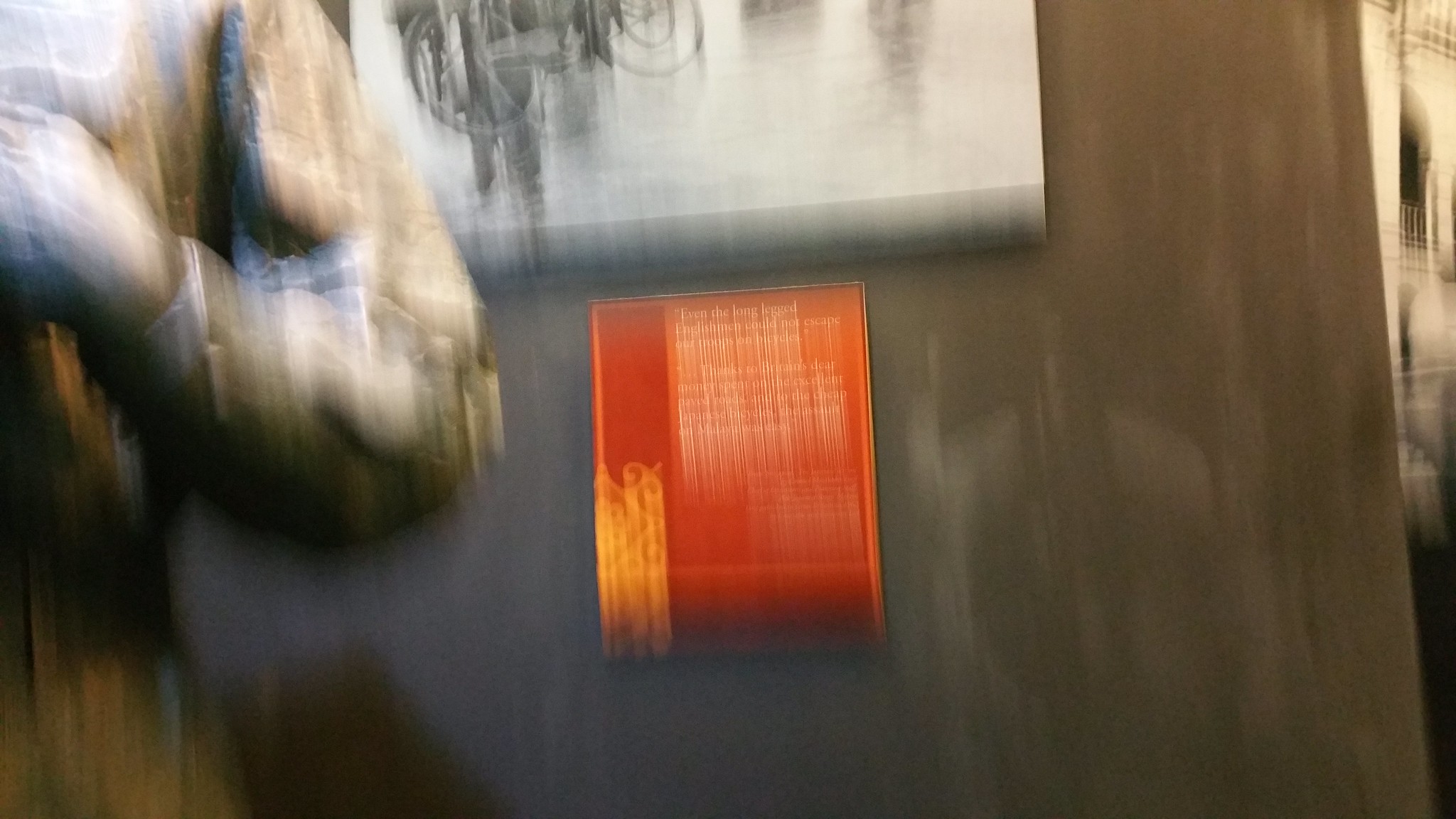The image appears to be a blurry photograph taken indoors, likely in a museum setting. The focal point of the image is a dark wooden table at the center, upon which rests a bright red book adorned with orange trim along its edges. The book features an intricate yellow decoration on its left side that extends towards the center, forming swirls with a pointed front. Though the text on the book is largely unreadable, the first line appears to start with "even the long legend."

Above the table, affixed to a grayish-brown concrete wall, is a black and white piece of abstract artwork. The artwork, possibly created using charcoal or paint, features heavier strokes on the left and lighter wisps towards the right. Directly beneath this artwork is a vertical, reddish-orange plaque bearing an insignia, possibly the museum's crest, with partially readable white text. The first line of this text also seems to reference "even the long legend." On the far left side of the image, a stone sculpture of a person is partially visible, identifiable by its gray and brown left arm, which appears to be clothed in long sleeves. The overall scene suggests the image was captured hastily, resulting in its overall blurred effect.